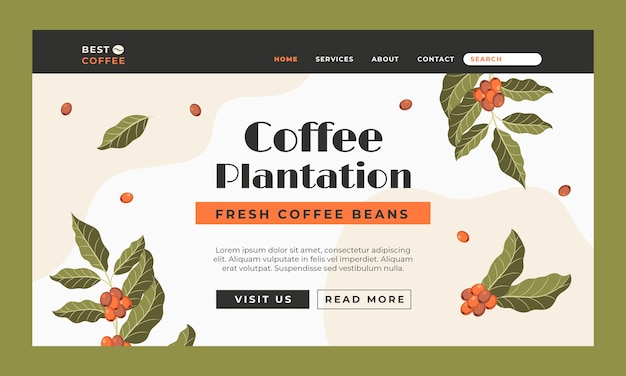The image depicts the landing page of a website designed to advertise coffee. The central section of the page is bordered by an olive-green trim, and within this rectangle, a black horizontal bar sits at the top. In the upper left of this bar, the words "Best Coffee" are prominently displayed, with "Best" in white and "Coffee" in orange. To the right, the navigation menu includes the links "Home" (in orange), "Services" (in white), "About," and "Contact," followed by a search bar.

Below the navigation bar, large text reads "Coffee Plantation," with "Fresh Coffee Beans" emphasized in black text against an orange rectangle. The main content is adorned with images of green leaves and red beans, illustrating coffee plants. Some leaves and beans are shown floating above the main images, adding a dynamic feel. Towards the bottom of the page, there is placeholder text in Latin ("Lorem Ipsum"), and it is flanked by two call-to-action buttons: "Visit Us" on the left and "Read More" on the right. The background of the image is primarily white.